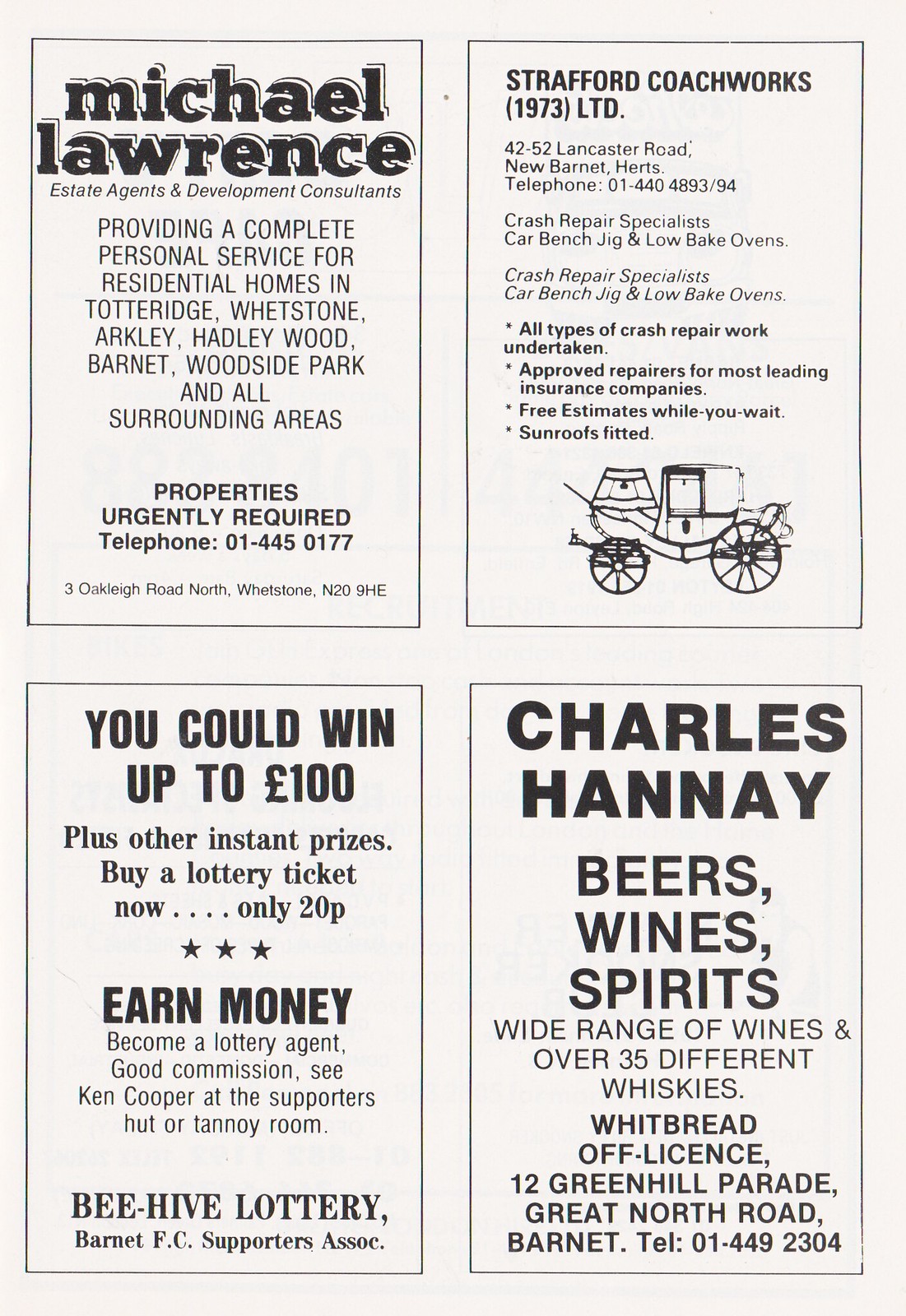The image showcases four vintage business advertisements, neatly arranged in a 2x2 grid with a small space in between each. Each ad is printed in dark lettering on a white background. The top left ad features Michael Lawrence in bold, 3D-type font, offering a complete personal service for residential homes in Totteridge, Whitestone, Arkley, Hartley, Wood Barnet, Woodside Park, and surrounding areas, with a call for urgently required properties. The top right ad is for Stratford Coachworks Limited, with detailed information about repairing coaches and all types of crash repair work. Below this ad is an old-fashioned illustration of a coach. The bottom left ad advertises a lottery by Beehive Lottery, promising potential winnings of up to 100 pounds and other instant prizes, with an encouragement to buy a ticket for 20 pence and earn money as a lottery agent. The bottom right ad is for Charles Hannon, prominently featuring "beer, wines, and spirits" in bold, followed by details about offering a wide range of wines and over 35 different whiskeys, located at 12 Green Hill Parade, Great North Road, with the phone number included. All four ads have varying font sizes and styles to emphasize the most important information.